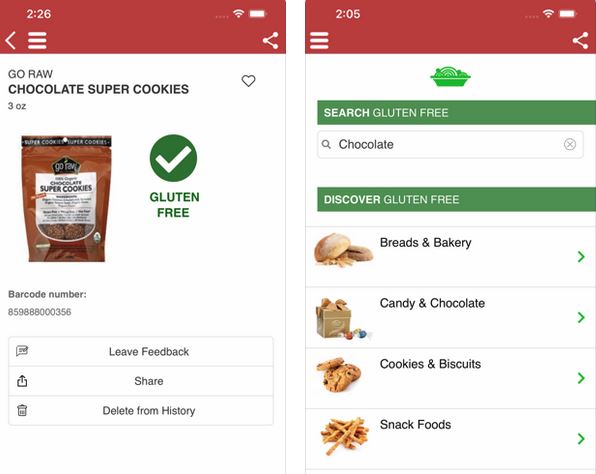This is a detailed caption for the described set of two screenshots from a person's cell phone:

---

**Set of Two Screenshots from a Cell Phone with Red Banners**

*Left Screenshot:*
The left screenshot features a red banner at the top with the number 226 prominently displayed. Below, the text "Go Raw Chocolate Super Cookies, 3 ounces" describes the product. A photograph of a brown bag containing the cookies is centered on the screen, with a clear section at the bottom of the bag revealing the cookies inside. Adjacent to the product photo, a green circle with a white check mark signifies the item's gluten-free status. Further information includes a barcode number, "859-888-000-356," and options to "Leave feedback," "Share," or "Delete from history."

*Right Screenshot:*
The right screenshot has a similar red banner at the top, marked with the number 205. It displays a search result for the term "gluten-free," specifically focusing on "Chocolate." Under the categorization "Discovered gluten-free," several sections are listed with corresponding images:
- "Breads and bakery" next to an image of two loaves of bread.
- "Candy and chocolate" featuring a brown box with wrapped truffles at the base, one truffle in a red wrapper and another in a green or blue wrapper.
- "Cookies and biscuits" accompanied by an image of three chocolate chip cookies.
- "Snack foods" with an image of a pile of pretzels.
The product images are all taller than they are wide. There are no people, animals, plants, flowers, or trees present in any of the images.